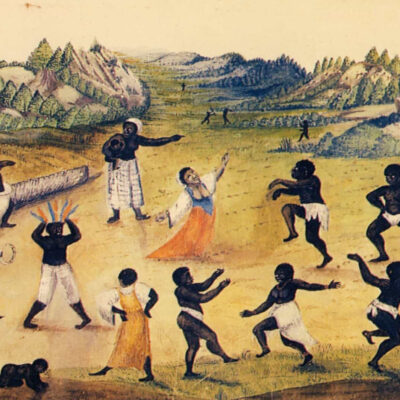The image is a scan of a detailed painting that depicts a vibrant celebration in a mountainous field. Central to the artwork is a light-skinned woman with a black afro, clothed in a distinctive dress featuring a blue torso, an orange skirt that extends past her feet, and white long sleeves. Surrounding her are about a dozen dark-skinned men and women, forming a circle as they dance exuberantly. The men are minimally dressed in white loin cloths, while the women are in white skirts or dresses, with one wearing a white dress accented with a gold apron. The field is bordered by rolling hills and mountains, some lush with greenery and others of a dark gray hue, adding depth to the scenic background. In the far distance, additional figures can be seen participating in the celebration, enhancing the lively and communal atmosphere of the scene.